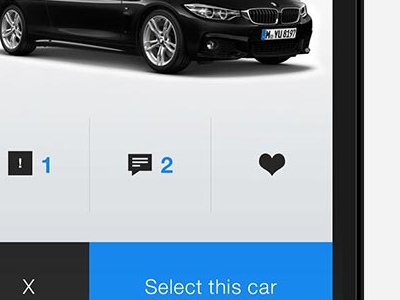The image appears to be a photograph of a tablet or laptop screen displaying a partially visible post that resembles an advertisement or social media post featuring a car. The photo has a nearly square rectangular format with a white strip running vertically along the far right edge, adjacent to a black strip that outlines the frame of the tablet or laptop screen. 

The primary focus of the image is the lower part of a black BMW, prominently showing its wheels, the bottom part of the doors, and the front section. The car is displayed on what seems to be a showroom floor, hinting at its pristine, polished condition. 

In the interface of the screen, there is an exclamation mark followed by the number '1', indicating perhaps a notification or alert. Below it, a comment section is indicated by a comment icon with the number '2', though the specific comments themselves are not visible. There is also a grey heart icon, suggesting that the post may or may not have been liked yet.

At the bottom left, there's a small grey square with a white cross inside it. To its right, a blue button with the text "Select this car" written in white is present, likely as a call-to-action for viewing or selecting the vehicle.

Overall, the image captures the essence of a digital interface, possibly an online advertisement or a social media post, with a focus on the featured BMW car.